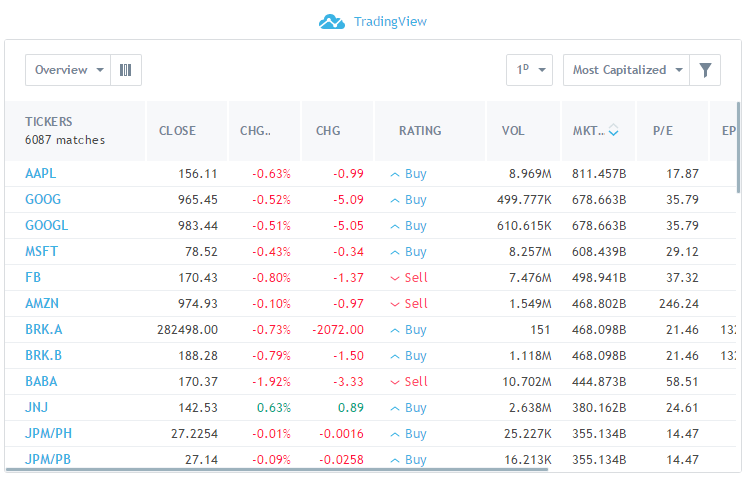The image appears to be a detailed screenshot from the TradingView platform. At the top, the TradingView logo is visible, indicating the source of the data. Dominating the image is a financial chart featuring a blue cloud with a white line running through it, symbolizing gains and returns, portraying profit and loss trends over time.

The interface is configured with filters specifying 'Overview' and 'Most Capitalized.' The results display 687 matches, although only 12 stock tickers are visible in the screenshot. These tickers include major companies such as Apple (AAPL), Google (GOOGL), Microsoft (MSFT), Facebook (FB), Amazon (AMZN), and others like Berkshire Hathaway Class A (BRK.A), Alibaba (BABA), Johnson & Johnson (JNJ), and JPMorgan Chase (JPM). Each ticker row displays crucial financial metrics such as the closing price, change (CHG) indicators, ratings, volume, market cap, price-to-earnings (PE) ratio, and additional data points. The layout is interactive, allowing users to scroll and reveal more information.